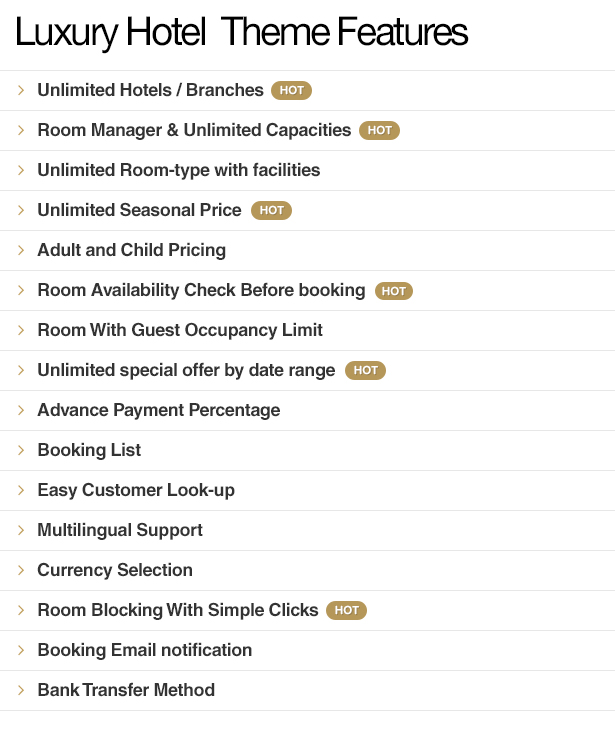This detailed caption describes the various features of a luxury hotel management system interface. 

---

The image showcases the main interface of a luxury hotel management system. The title 'Luxury Hotel Theme Features' is prominently displayed, emphasizing its significance with capitalized initials. Below the title, several key categories are listed, each equipped with interactive arrows for navigation to additional details or actions. The categories include: 

- **Unlimited Hotels/Branches**: An icon or 'hot button' is associated, indicating interactivity.
- **Room Manager and Unlimited Capacities**: Also accompanied by a hot button, suggesting further options or settings.
- **Unlimited Room Types with Facilities**
- **Unlimited Seasonal Pricing**: This category is also marked with a hot button.
- **Adult and Child Pricing**
- **Room Availability Check Before Booking**: Another hot button here implies real-time checks or live updates.
- **Room with Guest Occupancy Limit**
- **Unlimited Special Offers by Date Range**: Highlighted with a hot button, suggesting periodic promotions.
- **Advanced Payment Percentage**
- **Booking List**
- **Easy Customer Lookup**
- **Multilingual Support**
- **Currency Selection** 
- **Room Blocking with Simple Clicks**: A hot button indicates easy interaction.
- **Booking Email Notifications**
- **Bank Transfer Method**

Each category features a clickable arrow, providing a gateway to additional functionalities or subcategories. The design underscores user-friendliness and comprehensive control, ensuring efficient management for luxury hotel operators.